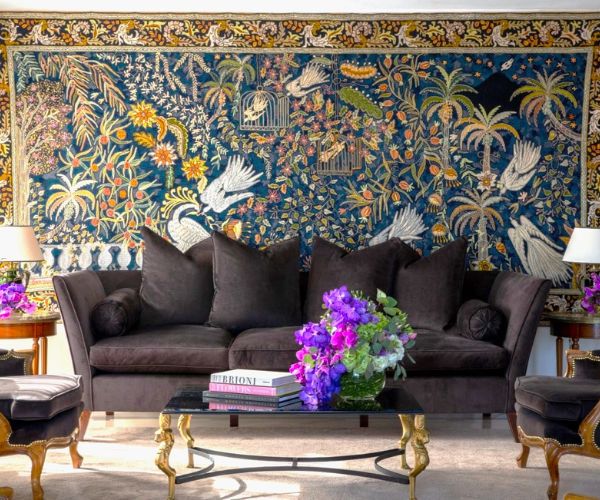This detailed photograph captures an intricately decorated living room. At the center, a dark-colored sofa, which might be either dark brown or grayish-black, stands out against a vibrant Persian rug hung on the wall. The rug is adorned with motifs of blue and gold, featuring white birds amidst palm trees.

The sofa is generously cushioned with four large back pillows and two smaller oblong ones. In front of it, there is an elegant glass coffee table with golden metallic legs, hosting a beautiful arrangement of purple, pink, and white flowers in a green planter. Beside the floral arrangement, three books are neatly stacked, one of which is titled "Brioni."

Flanking the sofa are two matching chairs with wooden Queen Anne legs, upholstered in the same fabric as the sofa. The chairs enhance the room’s classic aesthetic. On either side of the sofa, small round tables hold lamps with white shades and pinkish bases.

A beige rug lies beneath the furniture ensemble, adding warmth to the setting. Additionally, an end table hosts more purple and pink flowers, complementing the floral arrangement on the coffee table. This room showcases a harmonious blend of colors and textures, creating a sophisticated and inviting ambiance.